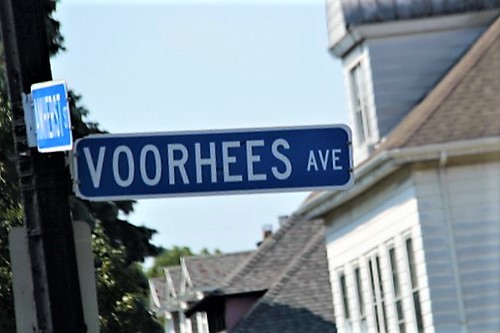The photograph captures an up-close view of a dark navy blue street sign with a white border, prominently displaying “VOORHEES Avenue” in large white text. The camera angle offers a side perspective, revealing an additional, unreadable blue street sign angled towards the viewer. Positioned on a white pole, the signs stand against a backdrop of a row of city-style houses. The foremost house features white siding, brown and gray shingled roofs, visible gutters, and a distinctive widow's peak, suggesting an attic space. Lining the street, the rooftops continue in similar dark brown and gray hues, punctuated by vertical windows and large, leafy trees. The image has a slight blur, contributing to a dreamy, almost nostalgic quality.